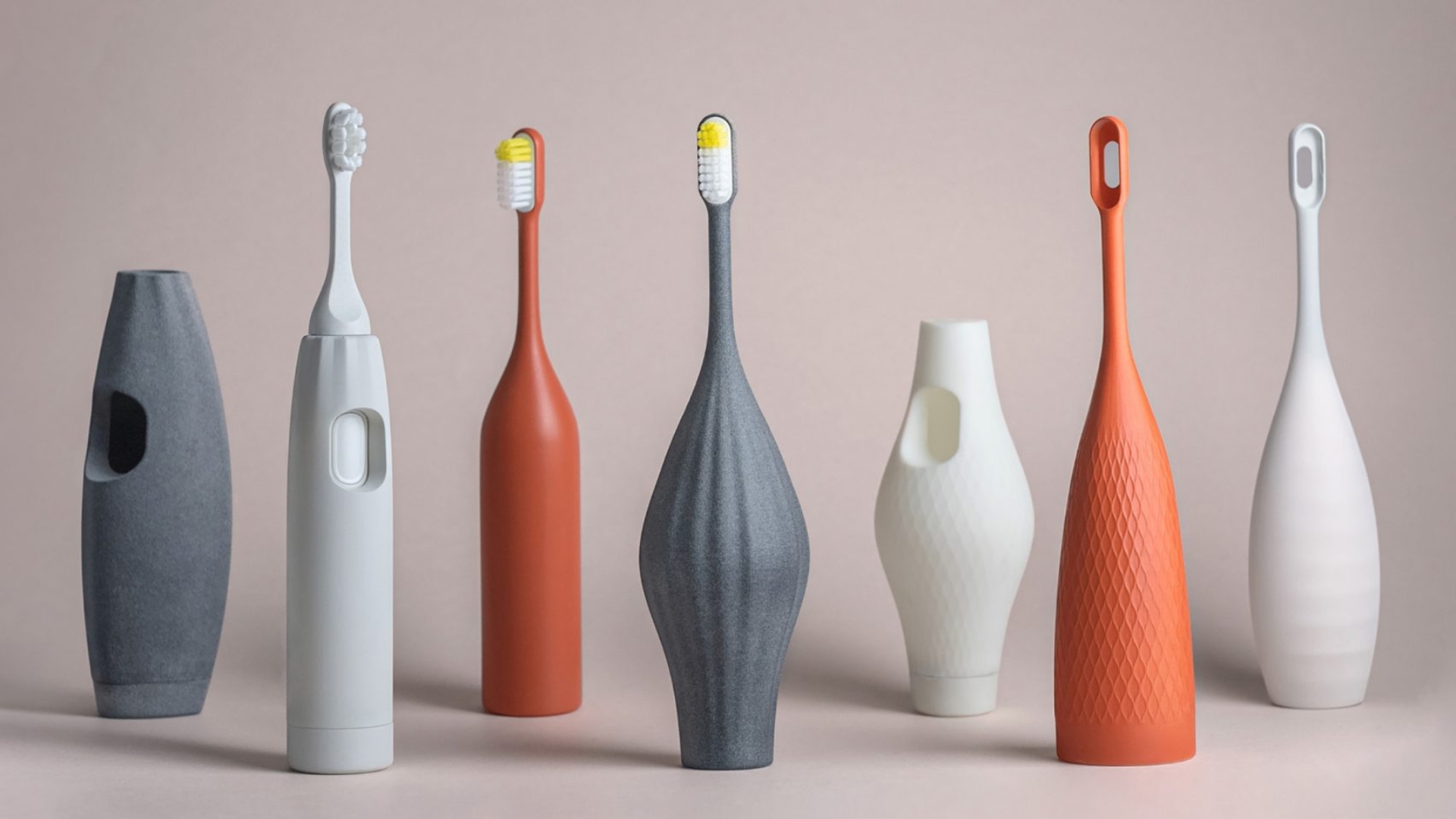This photograph features a collection of seven unique toothbrush designs arranged horizontally against a tan background. The items are distributed with three in the front row and four in the back row, alternating between being in the foreground and background. To the far left in the front row, there’s a gray, oval-shaped base with a hole on top. Following it, also in the front row, is a white, cylindrical-shaped holder containing a white toothbrush. Next, an orange holder shaped like a wine bottle, with white bristles tipped in yellow, stands prominently. The back row begins with another white holder resembling a shorter version of the gray base, featuring a hole on the top and side. Adjacent to it is an orange, bottle-like holder functioning as a toothbrush, showcasing white and yellow-tipped bristles. Another item in the front row, similar to a vase but also wider in the middle, is orange but without bristles. To the very right in the back row, a white holder with an empty slot where bristles would be completes the lineup, mirroring the toothbrush holders in the front row with alternating colors of white and gray. The arrangement and details captured suggest the toothbrushes are either inside an environment with no discernible indication of time of day.